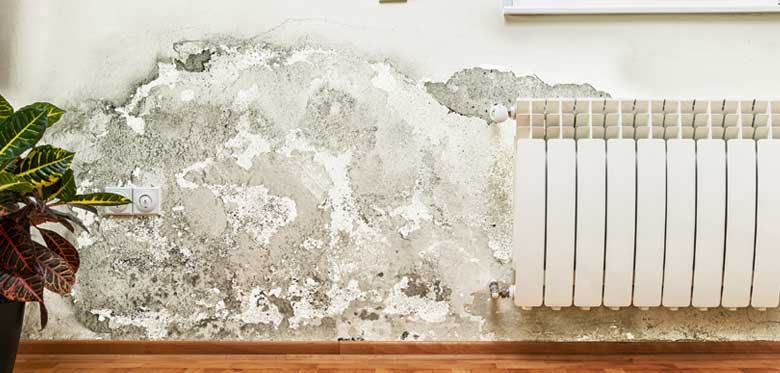This detailed, color photograph captures significant water damage on a once white stucco wall, now marred by mold and mildew. The damaged area spans approximately three by two and a half feet, revealing a mix of dark and light patches with rough, exposed cement. The lower part of the wall hosts white power sockets amidst the deterioration. Adjacent to this damaged section is a white steam radiator with a smooth metallic surface. The entire scene is bordered by a light brown hardwood floor. To the far left of the image, a black pot holds a plant, featuring a mix of green and reddish leaves. A ledge, possibly a window sill, is partially visible above the radiator, adding context to this indoor, likely residential, setting.